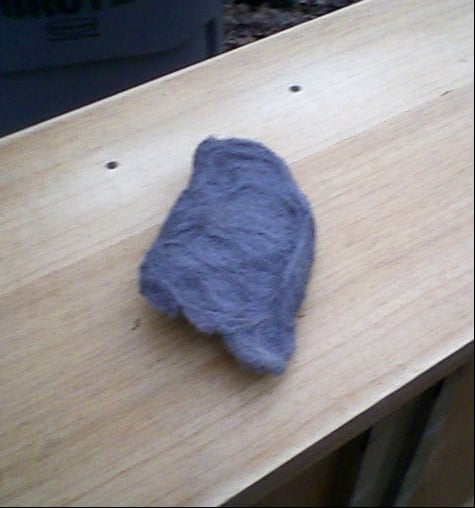In the center of the image, there's a bluish-gray object of an irregular, somewhat thick and fluffy texture, lying on a diagonally positioned piece of plywood. The object's material is ambiguous; it appears soft and could be fabric, lint, or even fur. The light brown plywood features darker grain patterns, with two small cut-out holes towards its top. The upper left-hand corner of the image reveals a handle attached to what looks like a cabinet, while the lower right-hand corner shows the rippled texture of a material resembling a sheet or curtain. The backdrop is not clearly defined, consisting possibly of a workshop or garage setting. The only colors discernible in the image are various shades of brown from the plywood, along with gray and purplish-blue hues from the unidentified central object. There is no text or writing present in the photograph.